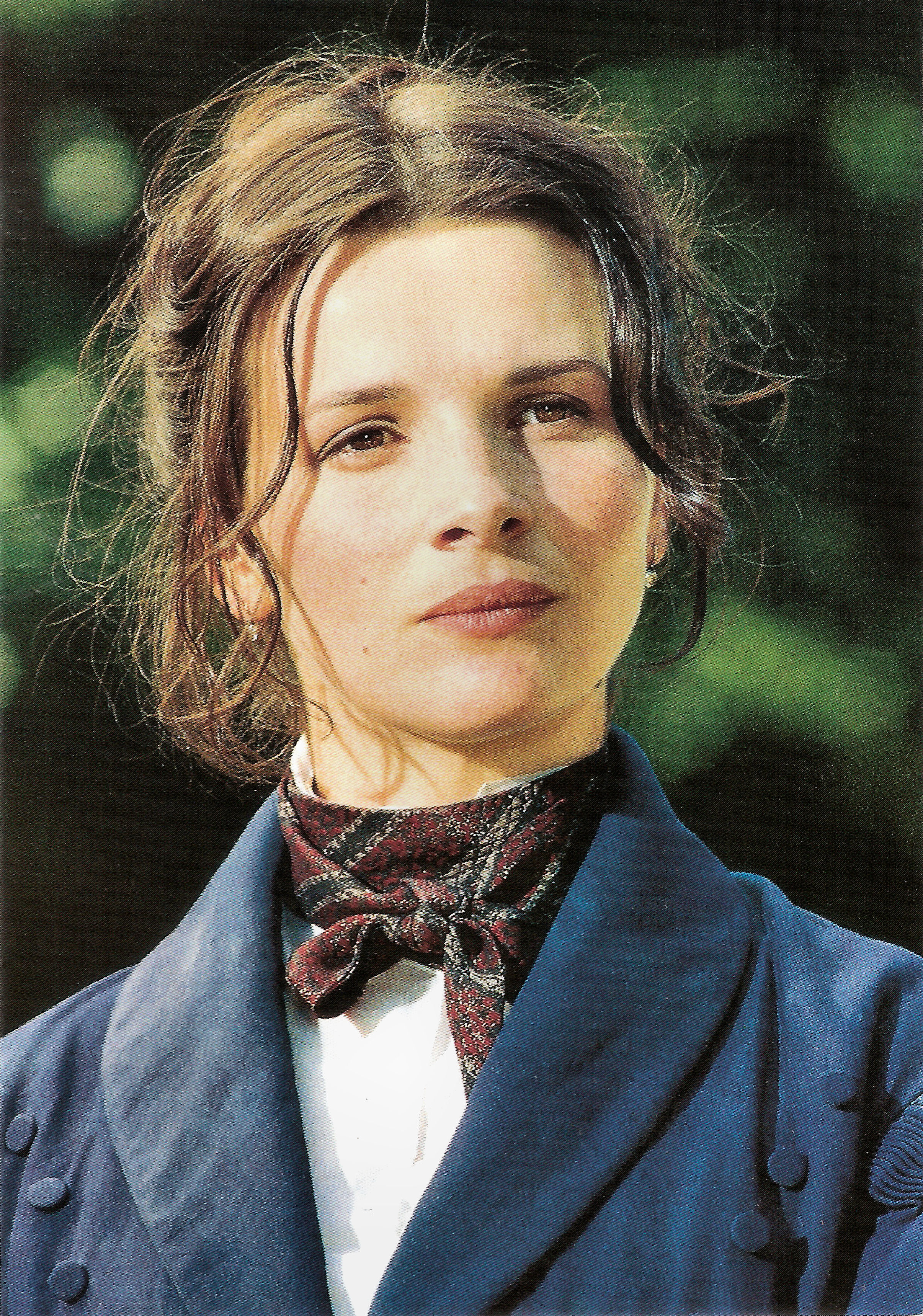This photograph captures a young lady, resembling an actress, adorned in a vintage Victorian-style ensemble. Her attire is a striking blue velvet blazer with pronounced large lapels and three visible buttons. A distinctive feature of her outfit is the purple and black bandana, tied around her neck where a bow would sit. She complements this with a white shirt underneath, giving a polished yet historical look.

Her brown hair is elegantly styled, flowing over her ears and partially up in a bun, while her face, illuminated by the sunlight, displays a neutral expression; she gazes intently to her left. The absence of lipstick and her natural brown eyes add to her captivating presence.

The backdrop hints at an outdoor setting with visible greenery, possibly trees, adding a serene touch to the photograph. This detailed and evocative portrayal suggests she might be part of a film or a similar period piece, capturing a moment of poised reflection.